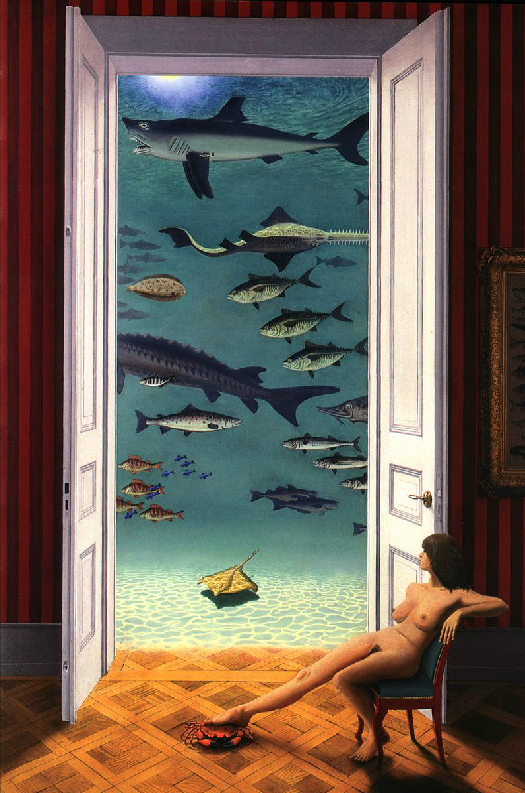In this highly detailed and intriguingly surreal painting, a nude woman with long, dark hair sits on a wooden chair adorned with a greenish-blue cushion, placed upon a parquet floor. Her left arm rests languidly over the back of the chair, while her right leg extends forward, intriguingly resting atop a crab, and her left leg tucks neatly under the chair. She gazes to her right toward a grand double door opened wide to reveal an underwater scene. The imposing, nearly ceiling-height white doors, decorated with rectangular and square designs, part to exhibit a vibrant aquatic world filled with diverse sea creatures, including a shark, a sawfish, a stingray, and various smaller fish. Above this watery tableau, the light source hovers, resembling either the sun or the moon above the water's surface. The scene outside is in stark contrast to the elegant room she resides in, characterized by vertical red and burgundy striped wallpaper and a baseboard. To the right of the doors hangs a large framed photo, its subject obscured from view. The overall composition creates a striking interplay between the serene domestic interior and the vibrant, dynamic marine life beyond.